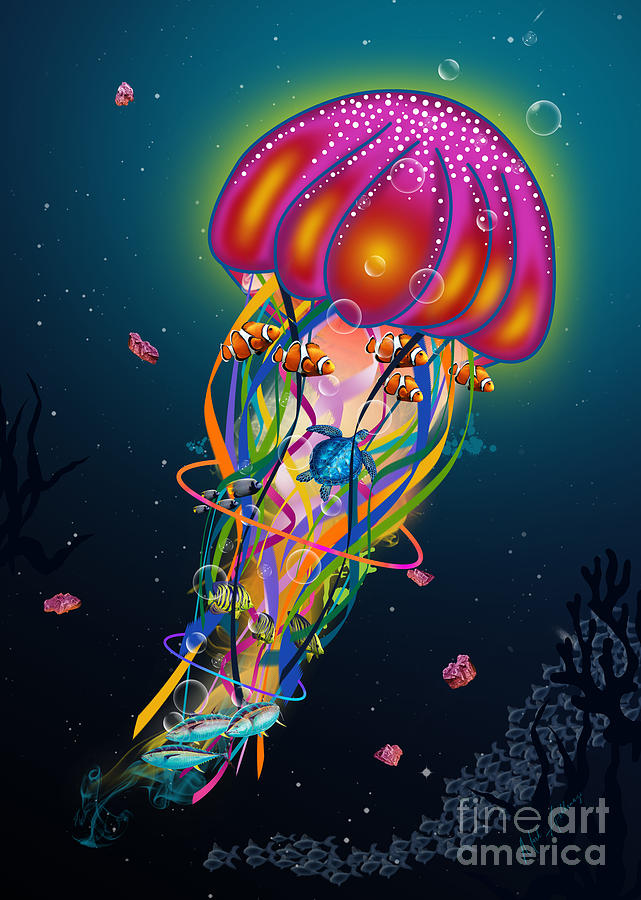This is an imaginative illustration of a jellyfish, prominently featured against a teal or bluish-green background that evokes the ocean depths. The jellyfish itself is depicted with a glowing pink and orange bell, adorned with white dots and intricate blue details. Cascading from its top are ribbon-like tentacles in a spectrum of vibrant colors: blue, green, yellow, red, and pink. Entwined among these tendrils are an array of marine creatures, including orange and white-striped clownfish, a small blue turtle, and several blue fish, adding a touch of surrealism to the scene.

Amid the jellyfish's tendrils, additional details like bubbles and patches of seaweed can be seen, along with some pink detritus. The top of the jellyfish emits a faint green glow, enhancing its otherworldly appearance. At the bottom right of the poster is a semi-transparent watermark reading "Fine Art America," with an underlay that could be interpreted as underwater foliage or a school of semi-translucent fish. The overall composition is artistically rendered, with a dreamlike quality that combines elements of realism and fantasy, resulting in a visually striking piece.